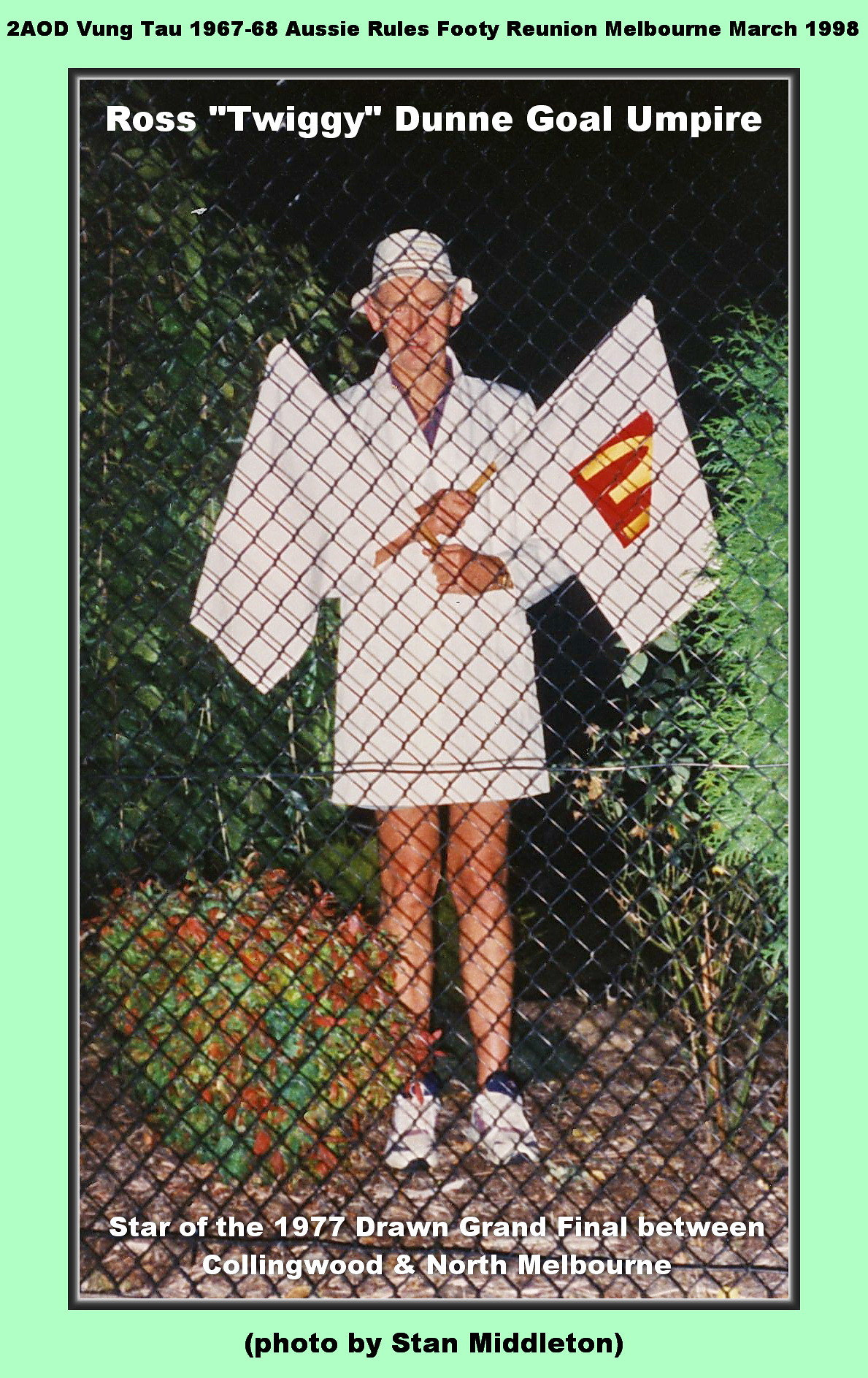This detailed photograph, set within a green frame, captures Ross Twiggy Dunn, a goal umpire, during the night. The older image shows Dunn in white shorts, a white knee-length jacket, and a white bucket hat, standing centrally against a dark background with green trees on either side. He holds two flags crossed over his chest, one plain white and the other displaying the McDonald's golden arches logo. The background indicates it's nighttime, with a chain link fence subtly visible. The top of the photograph reads "Ross Twiggy Dunn Goal Umpire," and at the bottom, "Star of the 1977 Drawn Grand Final between Collingwood and North Melbourne." Framing the image, the text at the top mentions "To A.O.D. Vung Tau 1967-68, Aussie Rules Footy Reunion, Melbourne, March 1998," while the bottom credits "Photo by Stan Middleton."